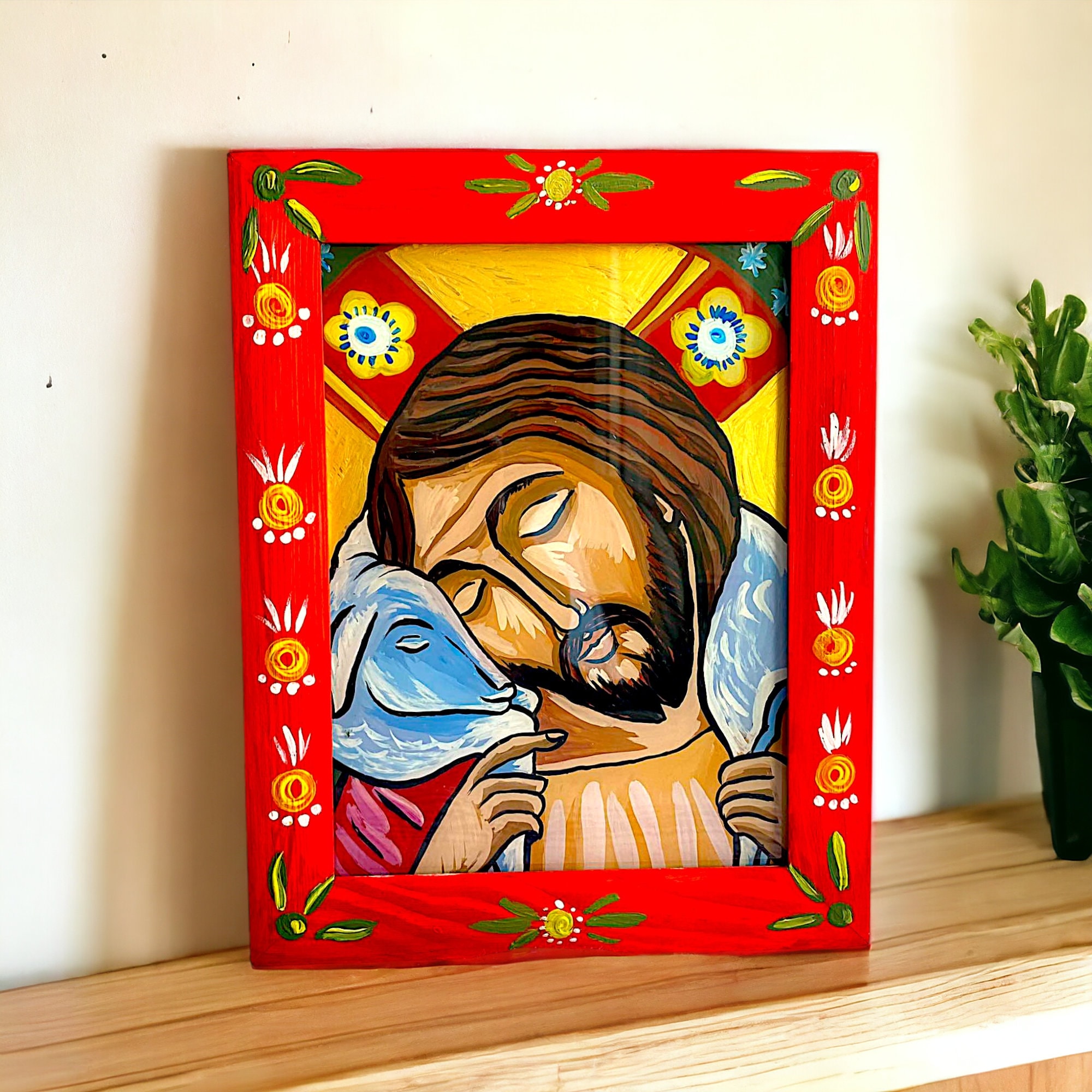The image captures a detailed and colorful scene centered around a picture frame with a vivid red wooden border. The frame is adorned with various painted designs: three green flowers at each corner, yellow flowers with green leaves at the top and bottom, and yellow pineapple-like patterns running down the sides. Inside the frame is a painting depicting a man, who appears to be Jesus, with long brown hair, tan skin, a mustache, and a beard. He is holding a blue lamb that rests at the back of his neck. The man's eyes are closed, as are the lamb’s. He wears a red shawl draped over his shoulders. The background of the painting is primarily yellow with a red floral pattern featuring yellow flowers with blue centers. The entire framed artwork is placed on a light brown wooden sill, and next to it on the right is a flower pot with green leaves. The wall behind the setup is white, providing a clean contrast to the vivid colors of the frame and painting.